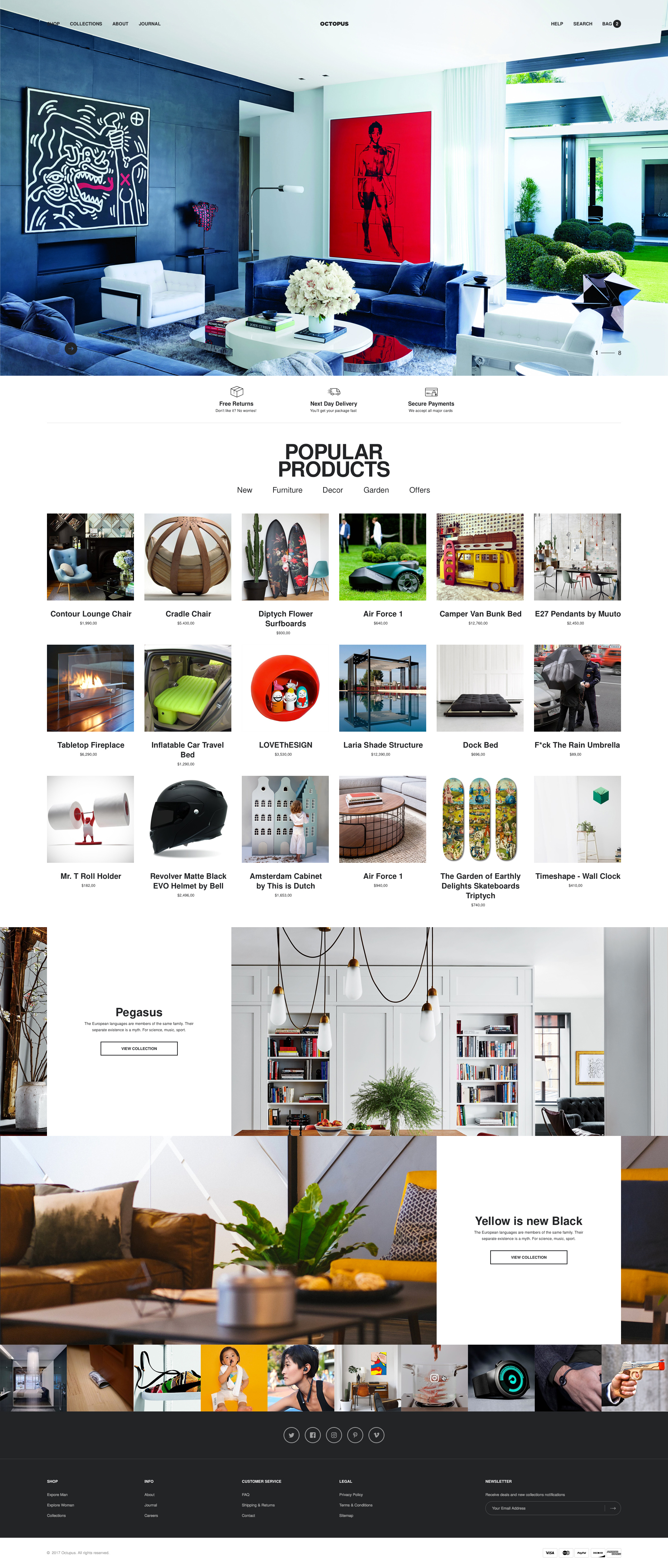A full-screen capture of a vibrant interior design website is displayed. At the top, there is a striking hero image featuring a room with a vibrant blue wall contrasted by a white wall adorned with a dynamic, bright red painting of a person in black silhouette. This sophisticated room arrangement includes two dark blue sofa seats facing each other, paired with two white chairs positioned opposite each other around a central white table. The table is embellished with a blue book that matches the sofas and a white flower pot. Through either a large window or an open door to the right, a lush interior garden or patio is visible, showcasing bright green grass and dark green bushes, adding to the room’s lively ambiance. 

Below this hero image are popular products, including a Contour Lounge Chair, a Cradle Chair, decorative flower surfboards, and an item presumably a robotic lawnmower named Air Force. Two more interior design images follow: one showcasing a lounge space with bookshelves and another living room area with the headline "Yellow is the New Black," likely discussing color trends and applications. The website's footer at the bottom of the page contains various informational links, providing further details about the site.